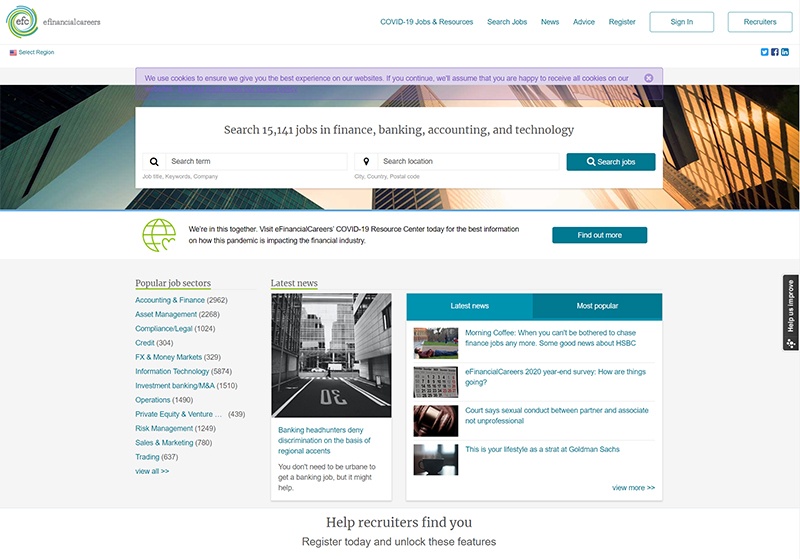The website screenshot is from eFinancialCareers, a prominent job site for finance professionals. In the upper left corner, the logo features "eFinancialCareers" and the initials "EFC" within a circle. Radiating outward from this are spiral patterns in shades of green and blue. 

On the upper right side, starting in the middle, the text "COVID-19 Jobs and Resources, Search Jobs, News, Advice, Register" is displayed. Further to the right, there are two buttons - one for signing in and another for recruiters, both outlined and text in green, set against a white background.

At the top center of the page, a purple strip announces: "We use cookies to ensure we give you the best experience on our website. If you continue, we'll assume that you are happy to receive all cookies on our site," accompanied by a circular icon with an 'X' for closing the message.

Below this strip, the page highlights a search bar with text: "Search 15,141 jobs in finance, banking, accounting, and technology," followed by fields for entering search terms, locations, and jobs. An important announcement below this reads: "We're in this together. Visit eFinancialCareers' COVID-19 Resource Center today for the best information on how this pandemic is impacting the financial industry," with a 'Find out more' button located on the right.

In the left column, there is a list of popular job sectors with corresponding job counts: 
- Accounting and Finance: 2,962
- Asset Management: 2,268
- Compliance and Legal: 1,024
- Credit: 304

The overall design is clean and professional, reflecting the site's focus on finance-related career opportunities.